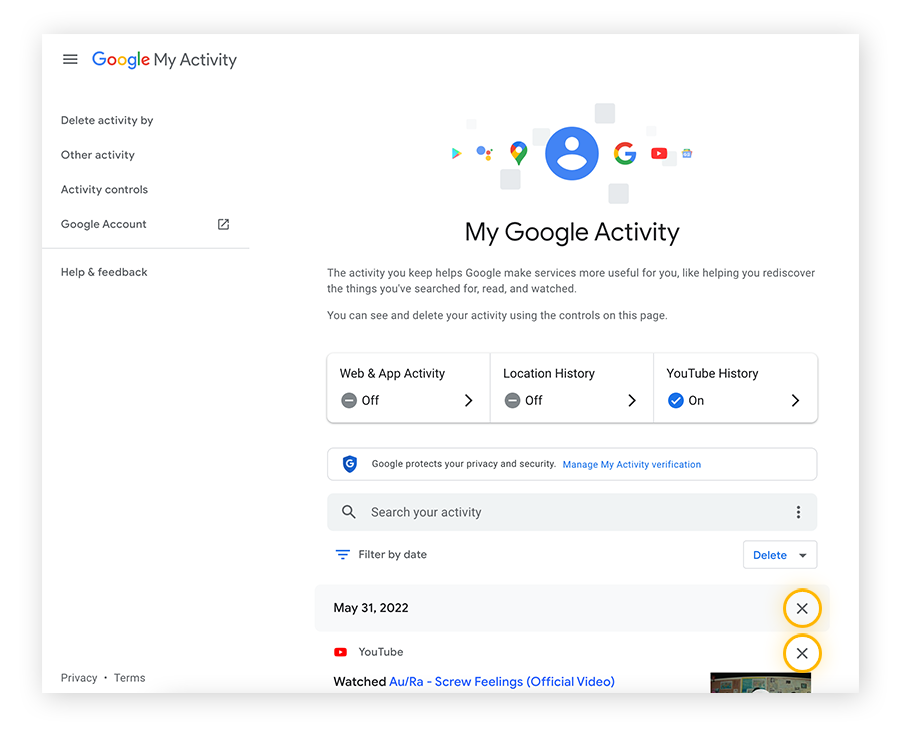The image appears to be a screenshot from a Google website, specifically the "My Activity" page. At the top left corner, the multicolored Google logo is prominently displayed next to the words "My Activity." On the left side, there is a sidebar menu that includes options such as "Delete activity by," "Other activity," "Activity controls," "Google account" (represented by a small square with an arrow inside it), and "Help and feedback," listed sequentially with a dividing line beneath the Google account option.

On the right side, the screen is headed by the text "My Google Activity," which is positioned above a series of icons representing various Google apps. These icons include the arrow symbol for the Play Store, the marker for Google Maps, the large "G" for general Google services, and the play button icon for YouTube.

The main section of the page explains that the activity you keep helps Google make its services more useful to you by assisting you in rediscovering past searches, reads, and watched content. It notes that you can review and delete your activity using the controls on this page.

Below this explanatory text is a bar divided into three sections:
1. "Web & App Activity" is labeled as "Off."
2. "Location History" is also marked as "Off."
3. "YouTube History" is indicated as "On."